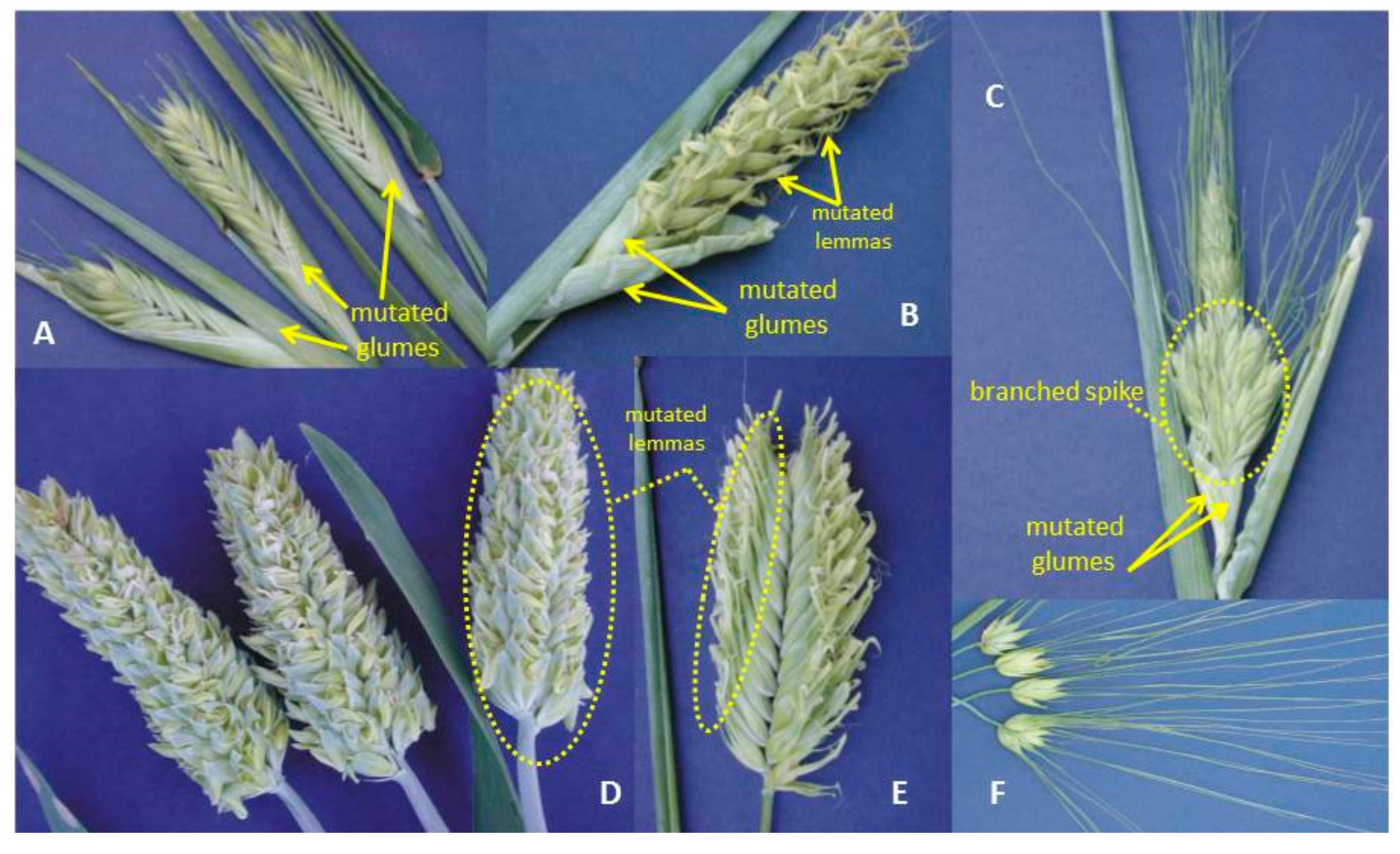The image is a detailed scientific composite consisting of six side-by-side labeled photographs (A, B, C, D, E, F) set against a blue background. Each photo highlights different stages and parts of wheat development, particularly focusing on mutations. Photo A displays three wheat heads with arrows pointing to the lower parts, labeled "mutated glumes." Photo B showcases a close-up of these mutations along with "mutated lemmas." Photo C features a branched spike and again emphasizes the "mutated glumes." Photos D and E provide even closer views of the "mutated lemmas," while Photo F shows four stalks aligned next to each other, further detailing the various wheat stages and mutations. The overall presentation aims to thoroughly illustrate the physical changes in wheat due to mutations, using precisely labeled and closely observed visual data.